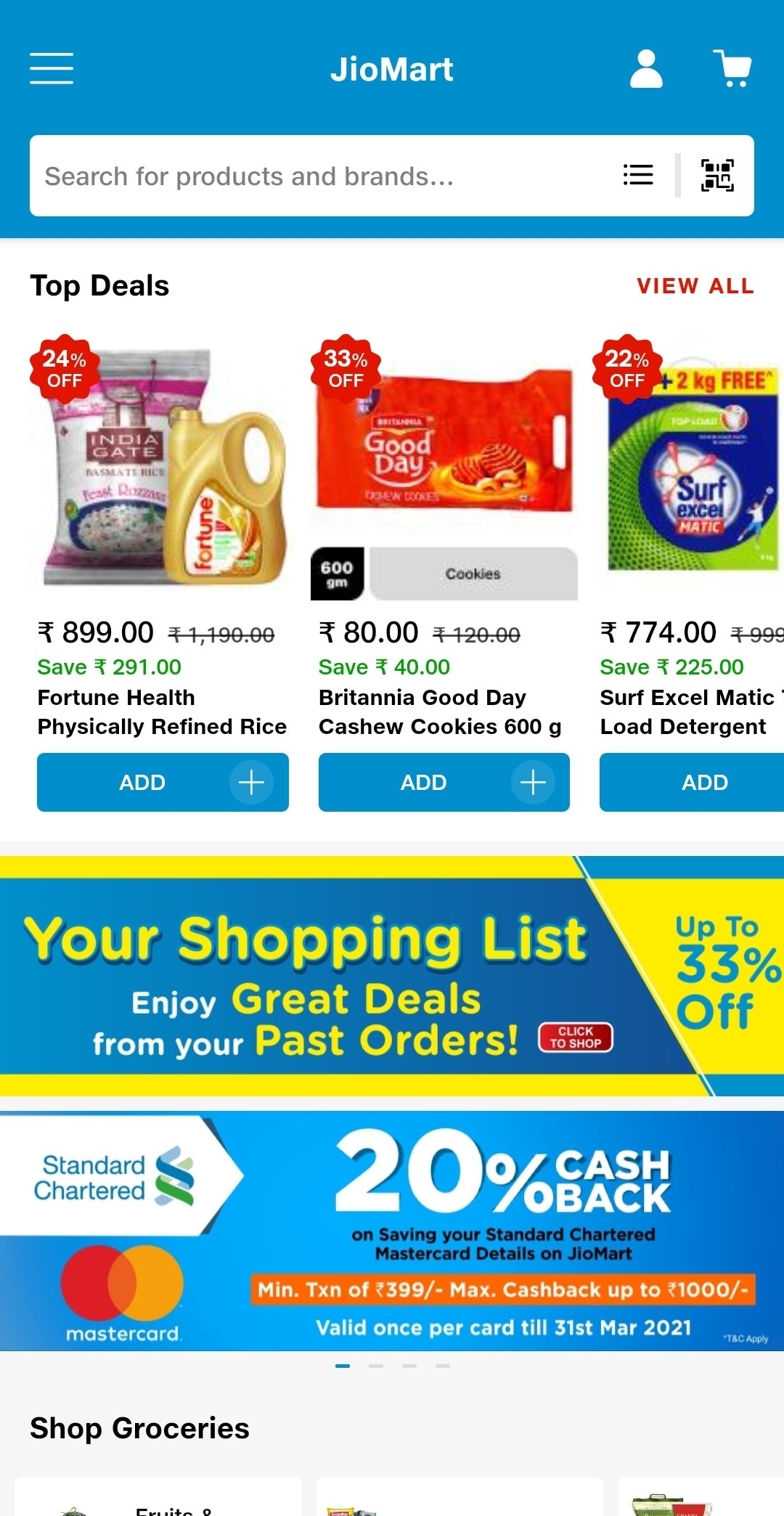This image appears to be a screenshot of a GyoMart mobile app interface. At the top, there is a blue rectangular banner displaying "GyoMart" in the center with a shopping cart icon to the right. Below this banner is a search bar with the placeholder text "Search for products and brands."

Directly underneath the search bar, there is a section titled "Top Deals" with a "View All" button on the right side. This section features three product graphics:

1. The first product is labeled "Fortune Health Physically Refined Rice," priced at $8.99, with a savings of $2.91. Above the product image, which shows a bag of rice, there is a "24% off" label. Below the image, there is an "Add" button.

2. The second product, situated in the middle, is "Britannia Good Day Cashew Cookies," priced at $80 with a discount saving of $40. The product image features a red bag of cookies labeled "Good Day," and it has a "33% off" label in the upper left corner. Below this product, there is also an "Add" button.

3. The third product, on the right, is a box of laundry detergent branded "Surf," priced at $7.74 with a savings of $2.25. This product is labeled "22% off," and an "Add" button is also placed below the image.

At the bottom of the screen, there are additional promotional advertisements. One highlights savings opportunities, titled "Your Shopping List," with a message suggesting, "Enjoy great deals from past orders, save up to 33% off." Another advertisement promotes MasterCard offers, stating "20% cash back valid once per card till 31st March 2021."